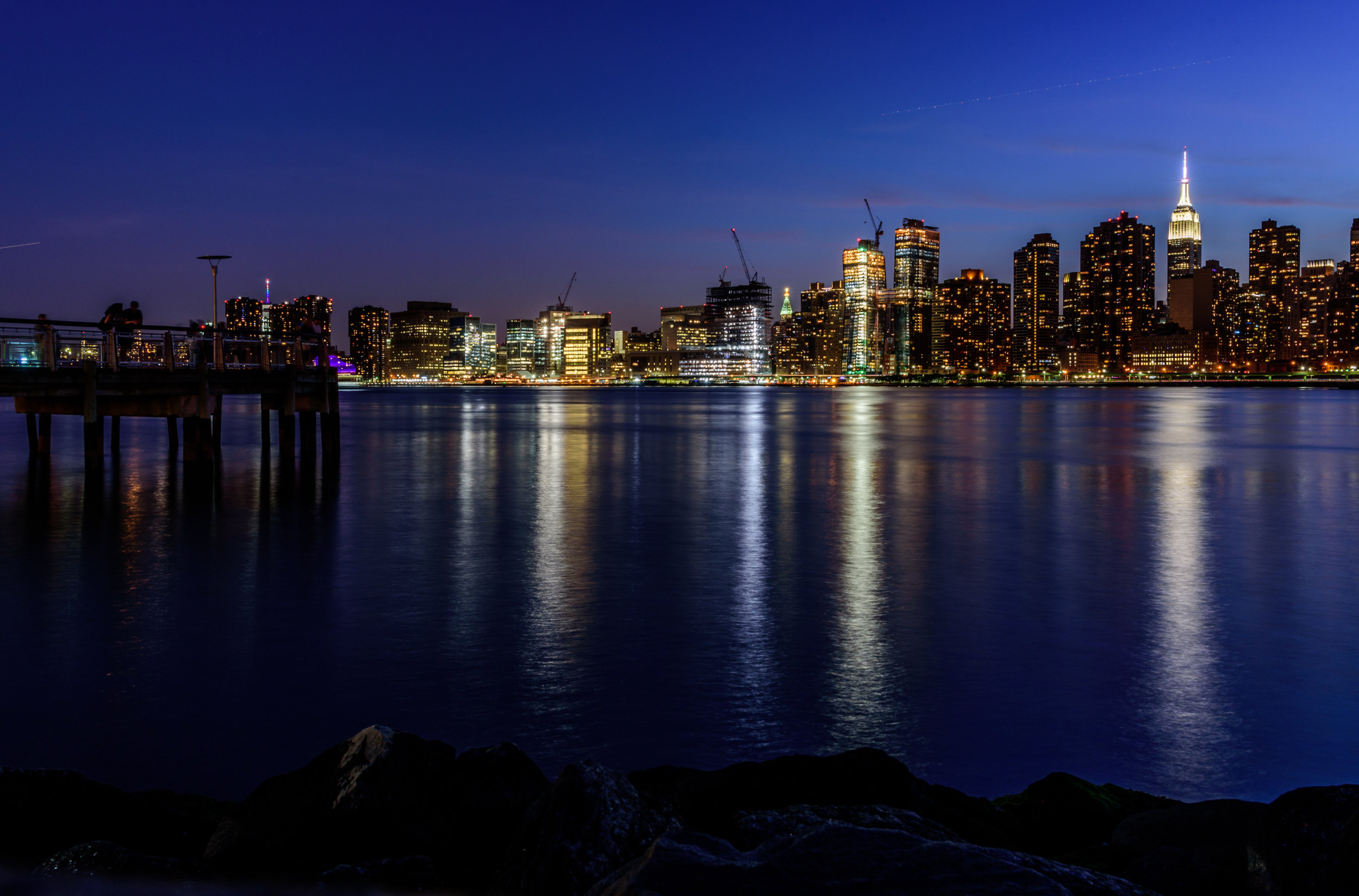In this nighttime cityscape photograph, the city stretches across the horizon, with its multitude of brightly lit skyscrapers reflecting on a dark blue, glistening body of water. A standout feature is a tall building with a needle-like spire, distinctly illuminated at its top floors, drawing the eye against the dusky night sky, which retains a bluish tint with a few scattered cirrus clouds. The viewpoint of the photograph is from across the river, where we stand on a cluster of rocks. To the left of the frame, a pier juts out, populated by people gazing at the brilliantly lit buildings across the water. The scene captures the bustling essence of the city at night, accented by the reflections of lights dancing on the tranquil river surface.